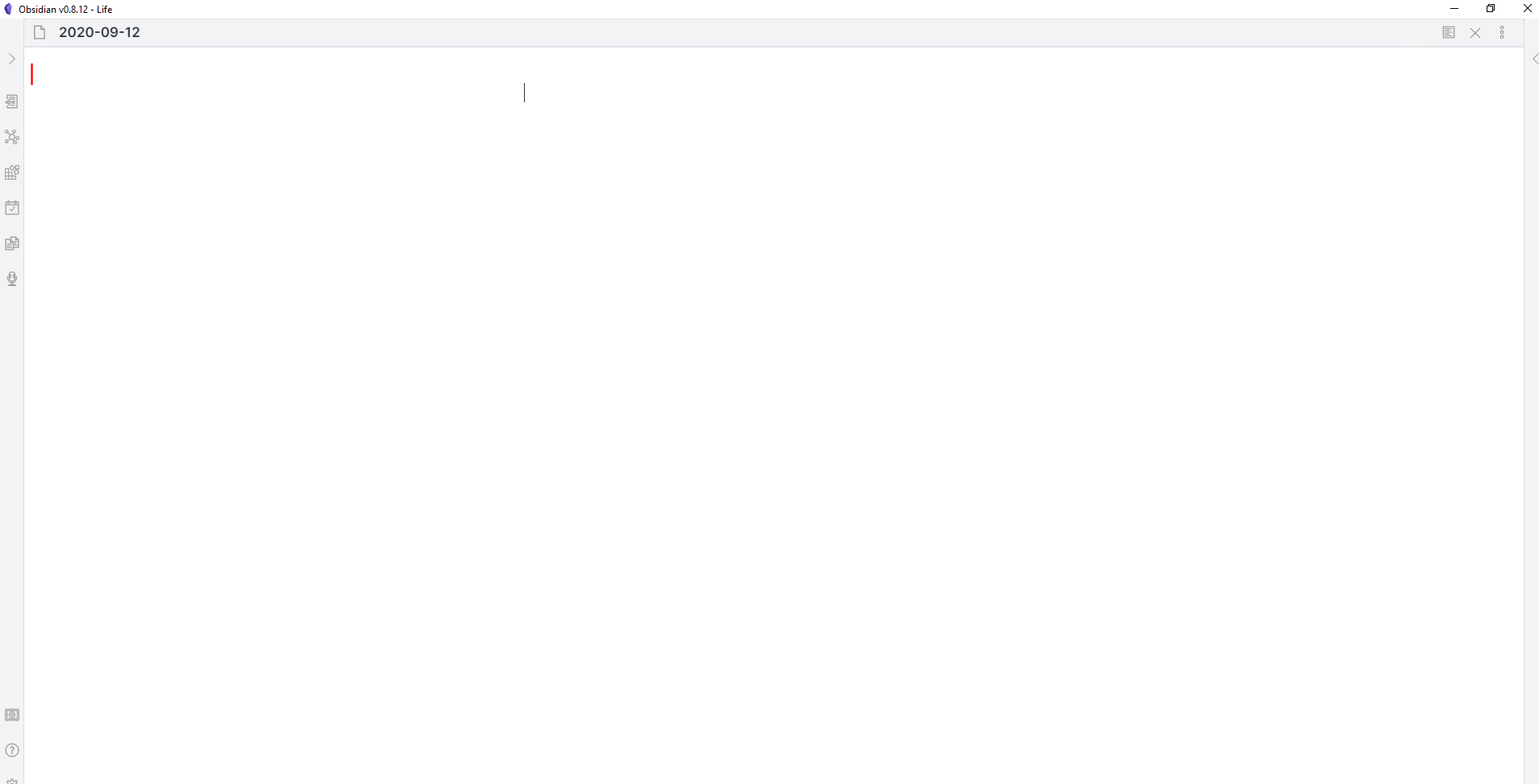This image captures the interface of a minimalistic application or website. The layout is presented with a primary focus on a vast, white, blank workspace that occupies the majority of the canvas. Encircling this workspace is a gray border, which serves as the application's menu bar.

The menu sections are positioned along the top and left edges of the interface. The top menu bar features, from left to right: a page icon followed by black text displaying the date "2020-09-12", and further to the right, a sequence of icons including a page, an "X", and a vertical ellipsis (three dots) suggesting additional functions or settings.

On the left-hand side, the vertical menu bar hosts several icons arranged from top to bottom: a page, an "X", another page, a folder, another page variant, and a microphone, each likely corresponding to different tools or features within the application.

Within the main white workspace, a solitary red vertical line cursor is positioned in the upper left corner, indicating a potential starting point for user input. Additionally, there is a black vertical line cursor located approximately one third from the left, situated on the same horizontal plane as its red counterpart, suggesting multiple points of interaction or selection within the blank canvas.